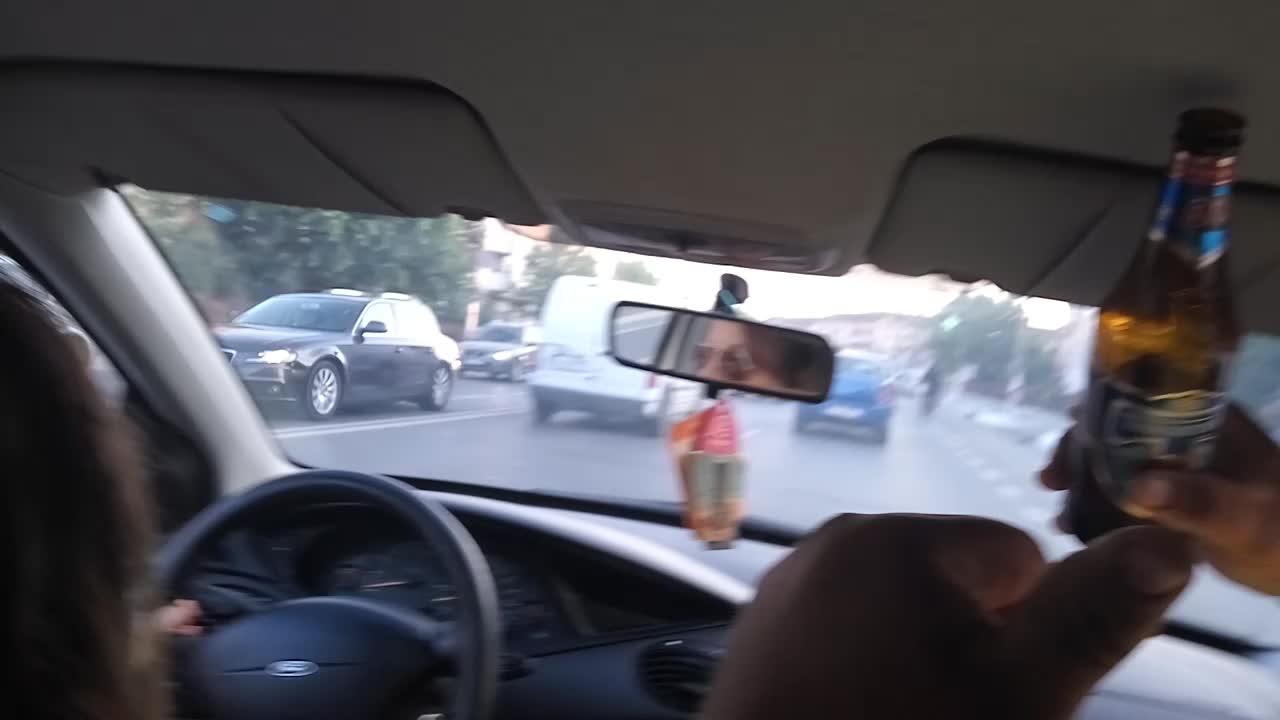In this photo, taken from the back seat of a car, a front-seat passenger is seen holding up a beer bottle in one hand and giving a thumbs up with the other. The shot is captured from directly behind the passenger-side seat, offering a clear view of the road ahead through the car's windshield. They are traveling on a three-lane road, positioned in the middle lane. Directly ahead of them is a blue car, while a white van is visible in the lane to the right. In the turn lane, designed to separate outgoing and incoming traffic, another car can be seen.

The reflection in the rearview mirror reveals the woman driver, wearing aviator sunglasses, with her long brown hair partially visible. Items hang from the rearview mirror, adding a personal touch to the vehicle's interior. Notably, the car is a Ford, as evidenced by the emblem on the steering wheel.